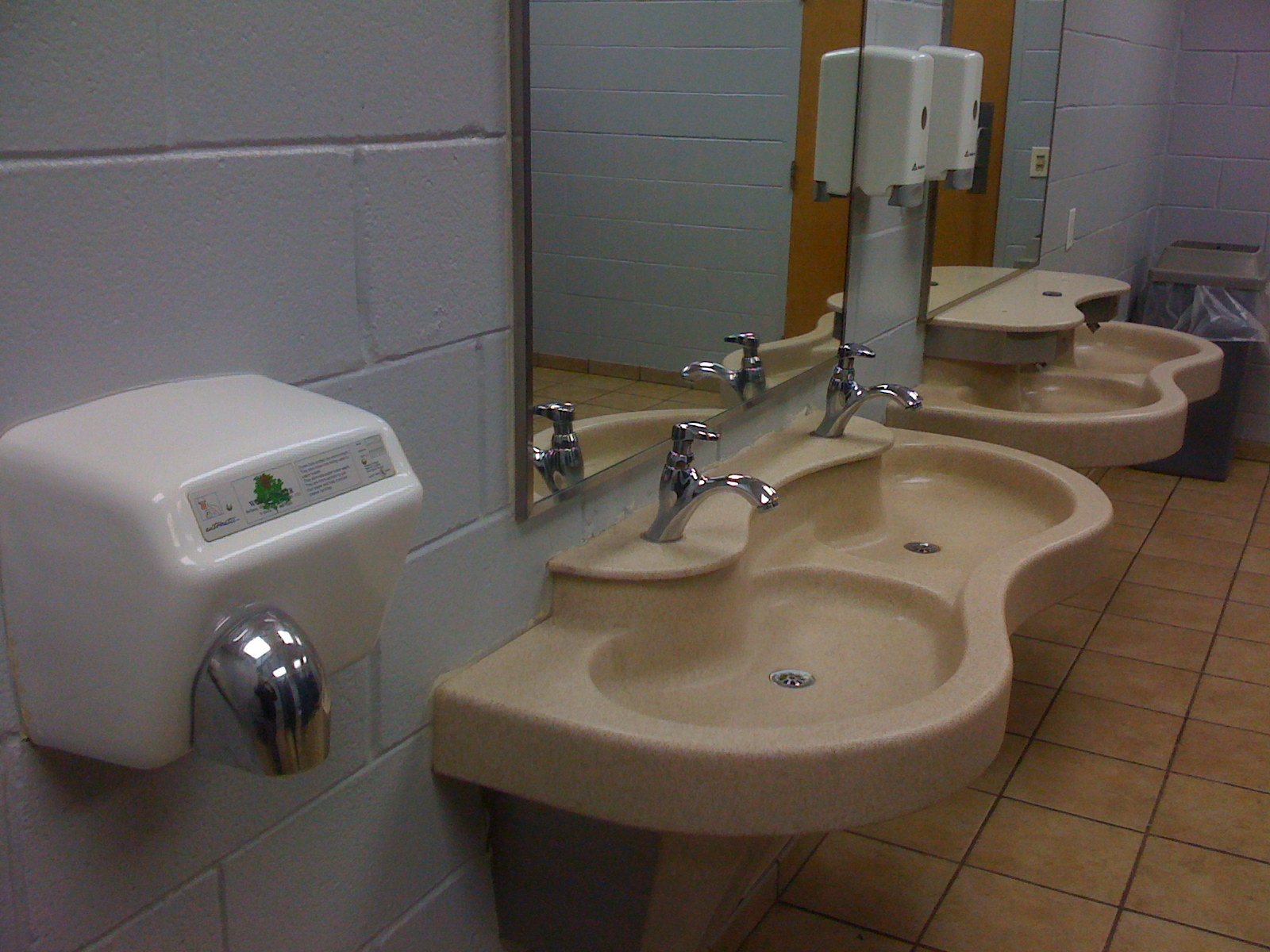The color photograph captures a public restroom featuring a white-painted cinder block wall. Mounted on the wall to the left is a white electric hand dryer with a chrome directional vent. The restroom has two curvilinear sinks made out of what seems to be Corian or a similar solid surface acrylic material, each resembling a peanut shape with two basins separated by a curve. The basins are paired, with each basin having its own arched chrome single-handle faucet. Positioned above each sink are wall-mounted mirrors and white and gray soap dispensers. The floor is covered with 12 by 12-inch tan tiles with black grout lines. In the background, a tall gray waste can with a flap lid, lined with a clear plastic bag, is visible. The restroom appears somewhat unclean.